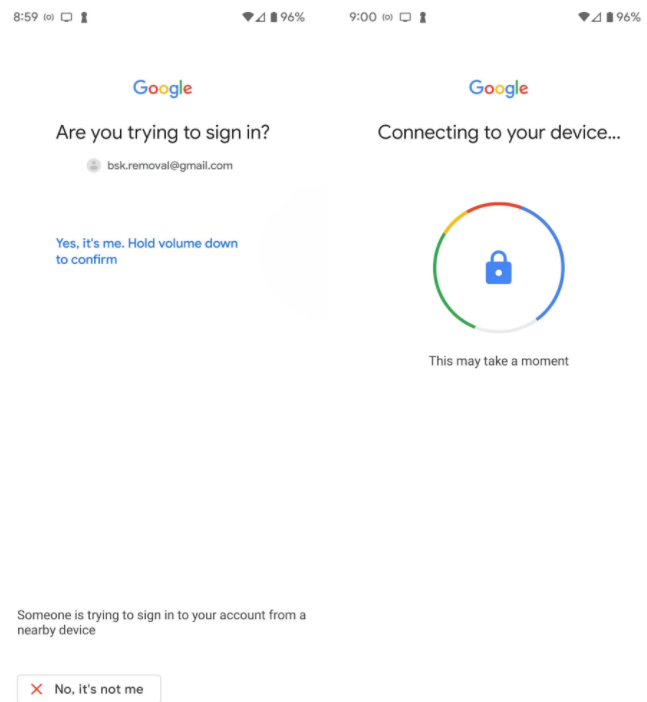The image features a white background with various elements related to a Google account sign-in verification process. 

On the left side, in grey font, it reads "859, 0 in a closed bracket, computer screen image, and keyhole". Next to it, there's an icon indicating a 96% battery along with a Wi-Fi symbol. This is mirrored again with text reading "9 o'clock, 0 in the brackets, computer image, keyhole, and 96% battery symbol with Wi-Fi."

Below, prominently displayed is the Google logo with its distinct colors: a blue 'G', red 'O', yellow 'O', blue 'G', green 'L', and red 'E'. Below the logo, in black font, it says "Are you trying to sign in?" followed by the email address "bsk.removal@gmail.com." 

To the right of this, another Google logo appears. Beneath it is the text "Connecting to your device." Returning to the left, there's a blue text saying "Yes, it's me. Hold volume down to confirm." 

On the right, there's a circular icon featuring colors red, blue, grey, green, and yellow, along with a blue padlock symbol with a white dot in the center. Below this, in black font, it says "This may take a moment."

At the bottom-left corner, in grey font, it mentions "Someone is trying to sign into your account from a nearby device." Next to this is a grey box with a red 'X' and the text "No, it's not me."